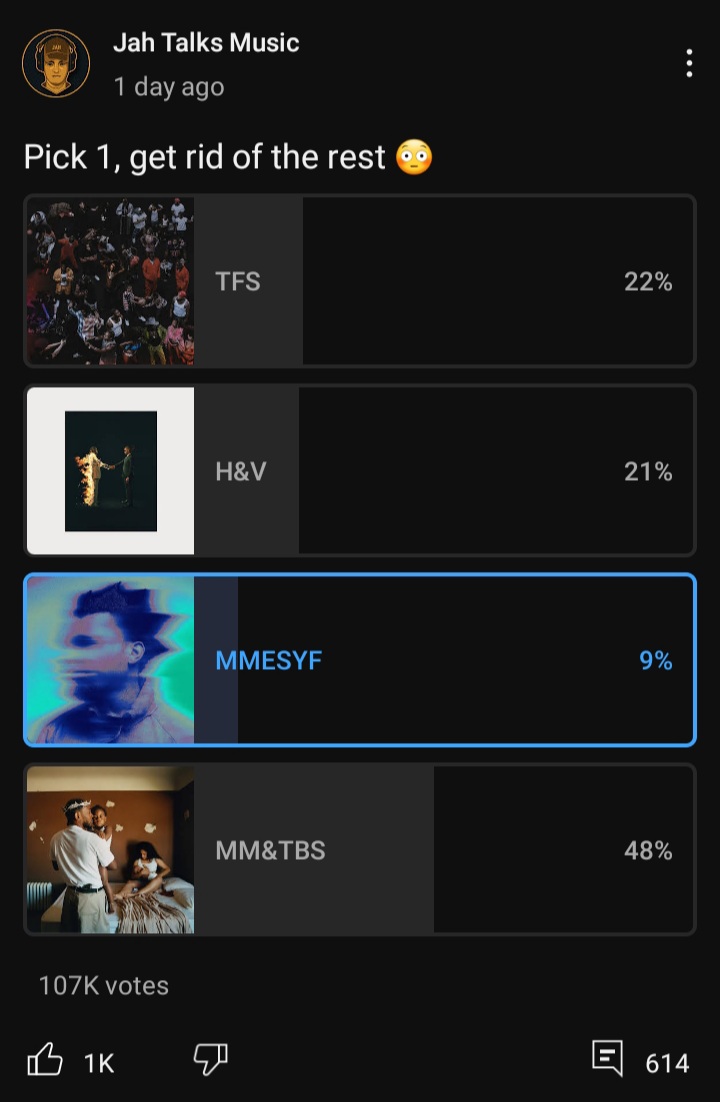The image features a black background with a gold emblem in the top left corner, depicting a person wearing a ball cap, sunglasses, and over-the-ear headphones. To the right of the emblem, there is white text that reads, "Ja Talks Music" followed by "One day ago." Further to the right, there is a caption that states, "Pick one, get rid of the rest," along with an emoji of a face with bulging eyes and an ellipsis.

Below the text, there are four indistinct thumbnails. Each thumbnail has accompanying text: the top one shows "TFS 22%," the second reads "H&V 21%," the third states "MMESYF 9%"—all of which are highlighted in light blue. The final thumbnail displays "MMMTBS 48%." Beneath these thumbnails, there is additional text that reads "107k votes, 1k likes, 614 comments," also in a light blue box.